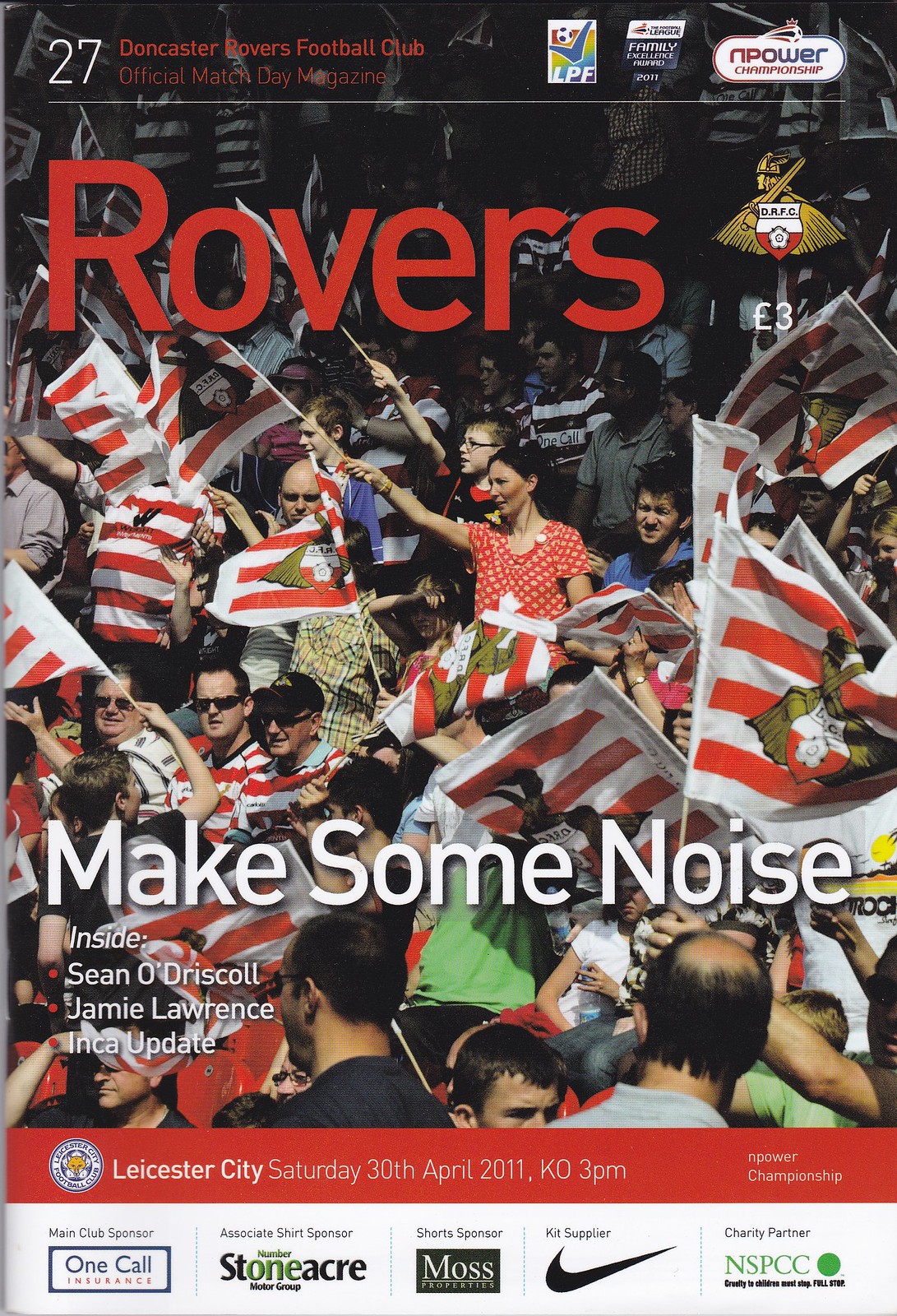The cover of the magazine titled "Rovers," Issue 27, showcases a vibrant, crowded stadium filled with fans holding flags adorned with red and white stripes, featuring a badge with an eagle and shield. The large red text at the top boldly announces "Rovers," while the caption beneath it proclaims, "Make Some Noise." The magazine prominently displays details such as "Doncaster Rovers Football Club Official Match Day Magazine" and highlights specific sections including "Inside: Sean O'Driscoll, Jamie Lawrence, Inca Update." The cover also provides crucial event details in a red banner at the bottom, stating "Leicester City, Saturday, 30th April 2011, Kickoff 3 PM." Sponsorship logos, including Nike, line the bottom, adding to the official look of the publication.